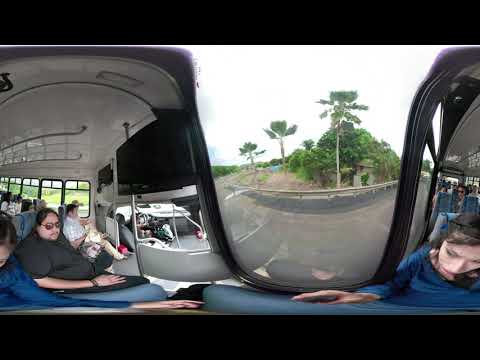This is a panoramic image taken inside a bus, likely during a relaxed trip, possibly in Hawaii, given the lush greenery and palm trees visible outside. The photo captures a variety of people seated in different positions due to the panoramic effect. On the left side, there is a large man with a white complexion, wearing sunglasses, a black shirt, and blue jeans. He has a goatee and is seated facing the right side of the frame. Next to him, a woman with dark hair wearing a dark blue shirt can be seen looking downward, her image also appearing on the right side due to the panoramic nature of the photo. The bus interior features white walls with black trim, and the sunlit scene outside the window showcases a clear blue sky, green trees, a road with a guardrail, and possibly an old building or a hill covered in vines and bushes. The atmosphere depicted is serene and joyous, reflecting a leisurely vacation vibe.